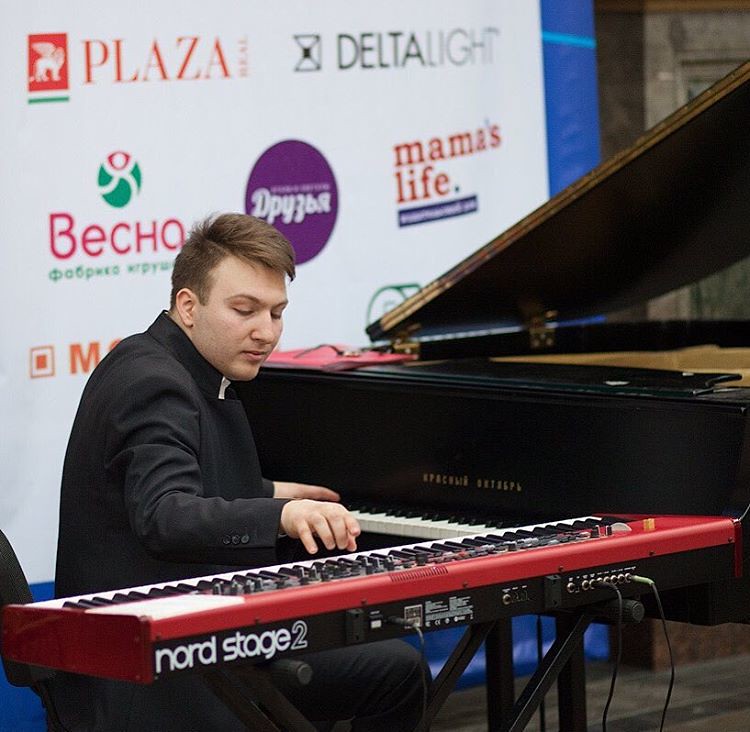A square photograph captures a young man immersed in a musical performance, set indoors against a backdrop of sponsor banners. The musician, donning a black jacket with the collar up, sits at an angled setup featuring a large black piano with its top open and a smaller red electronic keyboard to his right, marked "NORD Stage 2." He plays the piano with his left hand while simultaneously playing the keyboard with his right. His short brown hair and right ear are visible as he faces the instruments. Behind him, the sponsor banners display names such as Plaza, Delta Light—where "Delta" is bolded—Mama's Life, Beko in red, and additional text in various colors and languages. The photograph captures the concentrated energy of the musician at his dual-instrument setup, amid a scene indicative of a sponsored event.